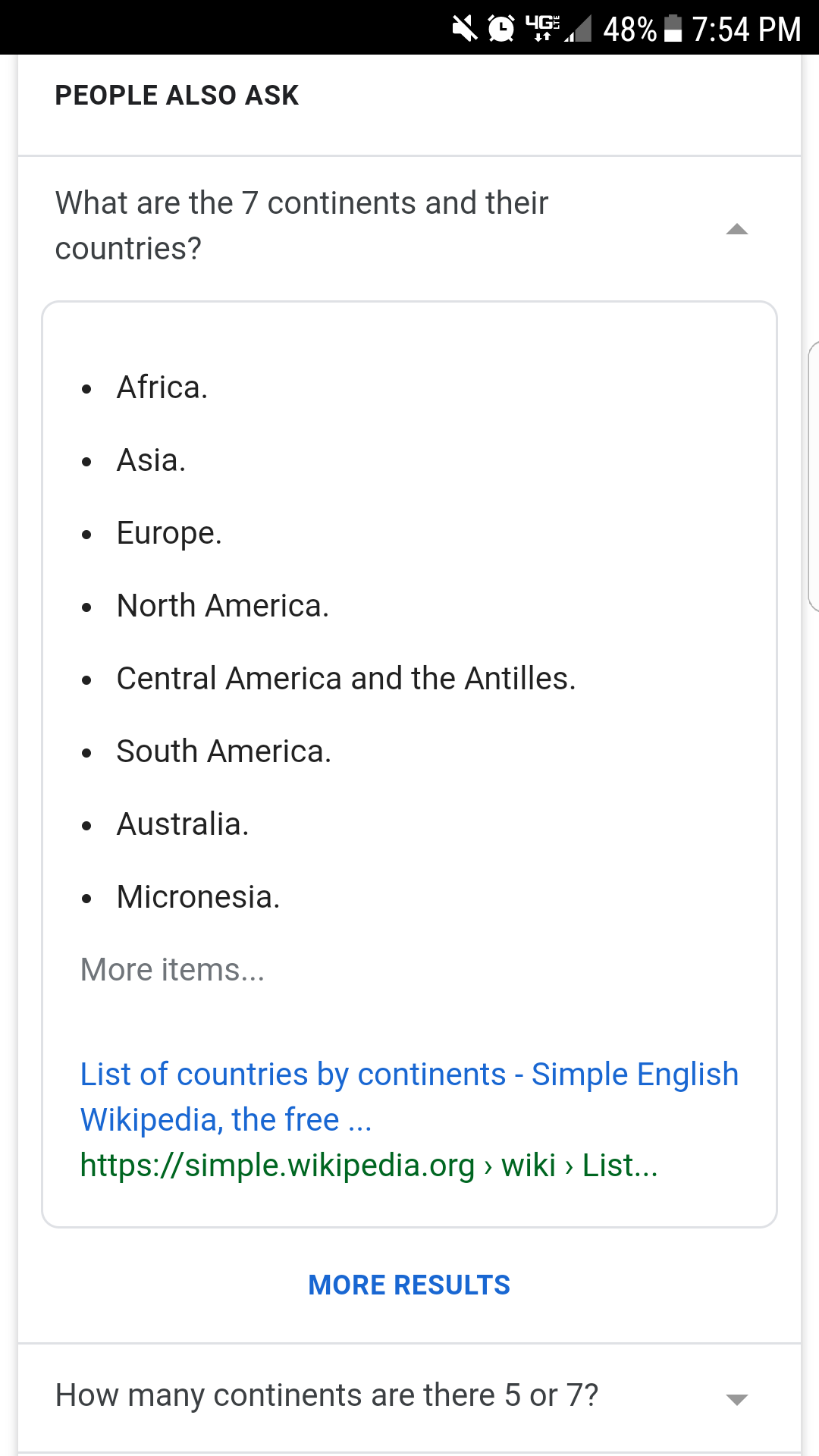The image depicts a search results page with a prominent "People Also Ask" section at the top. The highlighted question reads, "What are the seven continents and their countries?" Below this, a list of continents is provided: Africa, Asia, Europe, North America, Central America and the Antilles, South America, Australia, and Micronesia. Additionally, there is a snippet suggesting a source titled "List of countries by continents - Simple English Wikipedia, the free," although the rest of the text is truncated and not fully visible.